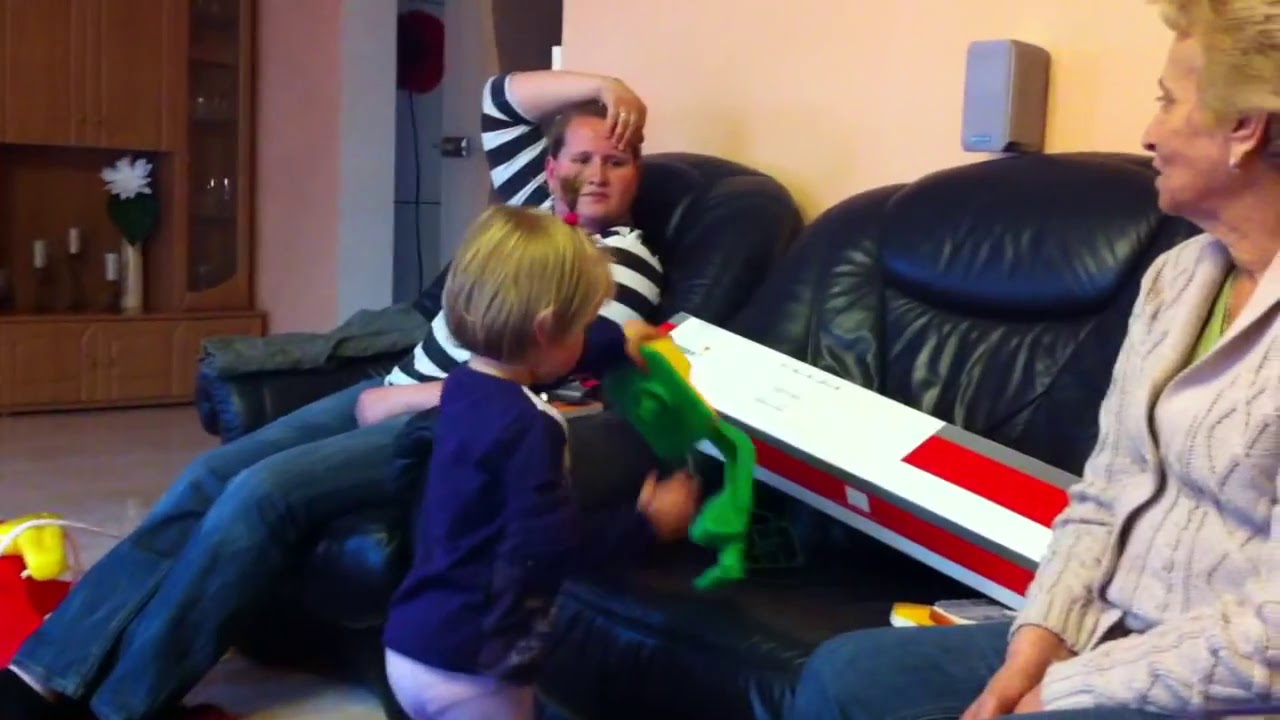The image captures a cozy living room scene with significant details focusing on the furniture and individuals present. The background features a wall with a wooden cabinet on the right, complete with shelves, and cabinets above and below. The main part of the image includes a black or blue leather sofa set against the wall. On the far right of this sofa is an older woman with short blonde hair, wearing a light-colored, possibly brown textured patterned or gray sweater over a lime green shirt, and blue jeans. She is sitting with her hands clasped between her legs, looking to her right towards the other individuals. To the left of her, closer to the front, is a large white box with red and gray stripes lying horizontally on the sofa.

Next to the box, a young child with short blonde hair, wearing a dark blue shirt and a diaper, stands facing the sofa and holding a green toy aloft. To the left of the sofa, a middle-aged woman with a round face, wearing a black and white striped shirt and blue jeans, sits with her right arm raised, her hand resting on her forehead, looking slightly to her right towards the camera. The room also features a doorway visible in the top left, adding to the home's inviting ambiance. The overall scene portrays a moment of everyday life, with each person seemingly engaged in their own activity amidst a well-furnished and warmly lit living room.